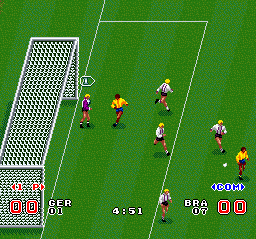This image is a low-resolution, square screenshot from an old and very basic computer or video game, possibly from a vintage console like a Game Boy or early Sega. It features a rudimentary representation of a soccer match between Germany (GER) and Brazil (BRA). 

The scene takes place on a green soccer field with darker green patches and white lines marking the boundaries and areas. On the left side is a goal post with a white net, where the game action is centered. A small, white soccer ball is visible near the goal. 

Players in the game are dressed in simplistic team uniforms: some wear yellow and blue, while others are in white and black attire; the goalkeeper on the left wears purple and black. At the bottom of the screen, the score is displayed in red for both teams, reading "0-0," signifying a tie. The match timer in the center indicates "4:51." Additional graphics show the letters "GER" and "BRA," with further notations like "01" and "07," likely relating to player statistics or team identifiers. This image captures an ongoing match, emphasizing the nostalgic, retro aesthetic of classic video games.